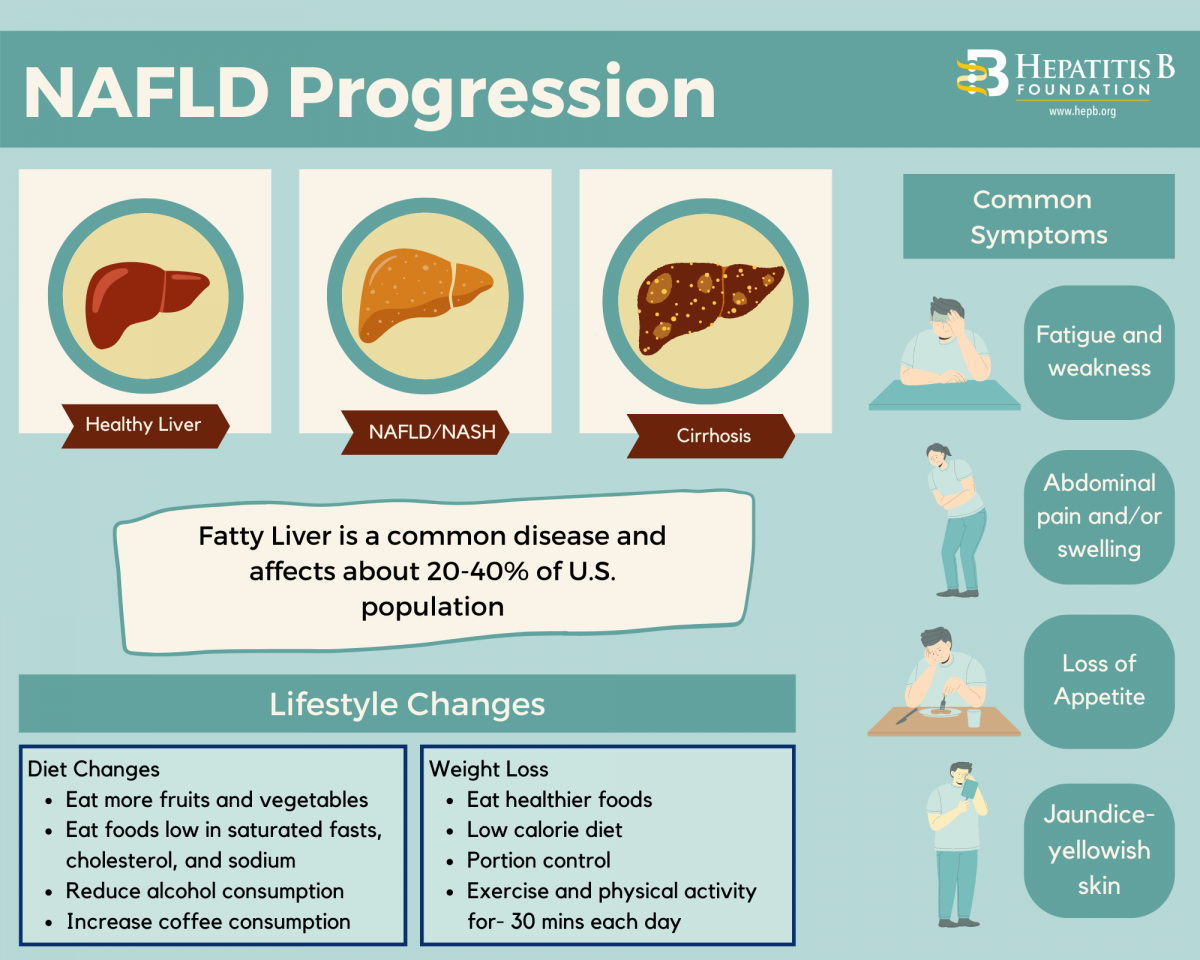**Poster for Hepatitis B Foundation: Understanding NAFLD Progression**

This detailed educational poster, presented by the Hepatitis B Foundation, focuses on the progression of Non-Alcoholic Fatty Liver Disease (NAFLD). The title, "NAFLD Progression," is prominently displayed at the top in bold white letters against a light blue background. The overall color scheme utilizes shades of light blue and teal for headers and accents.

The poster visually represents the various stages of liver health:
- **Healthy Liver:** Illustrated in a robust red color, indicating normal liver function.
- **NAFLD/NASH Liver:** Shown in a yellowish, spotted pattern, reflecting the fatty changes and hepatic inflammation associated with the disease.
- **Cirrhosis:** Depicted as a brown organ with yellow spots and white dots, signifying advanced liver damage with fibrosis and scarring.

On the right side, a vertical list highlights common symptoms of NAFLD with corresponding illustrations for clarity:
1. **Fatigue and Weakness:** Represented by an image of a tired individual.
2. **Abdominal Pain and/or Swelling:** Illustrated by a person clutching their abdomen in discomfort.
3. **Loss of Appetite:** Demonstrated by a figure disinterestedly staring at a plate of food.
4. **Jaundice (Yellowing of the Skin):** Shown by a character with a distinctly yellow complexion instead of their normal skin tone.

The lower section of the poster is dedicated to lifestyle changes that can help manage NAFLD. This section is divided into two categories, each set against a blue-bordered background with black text:
- **Dietary Changes:**
  - Increase intake of fruits and vegetables.
  - Consume foods low in cholesterol.
  - Reduce alcohol consumption.
  - Increase coffee consumption.

- **Weight Management and Activity:**
  - Emphasize weight loss through healthy food choices.
  - Follow a low-calorie diet with portion control.
  - Engage in regular physical activity, aiming for at least 30 minutes of exercise daily.

This visually engaging and informative poster serves as a comprehensive guide to understanding and managing NAFLD for patients and healthcare providers alike.